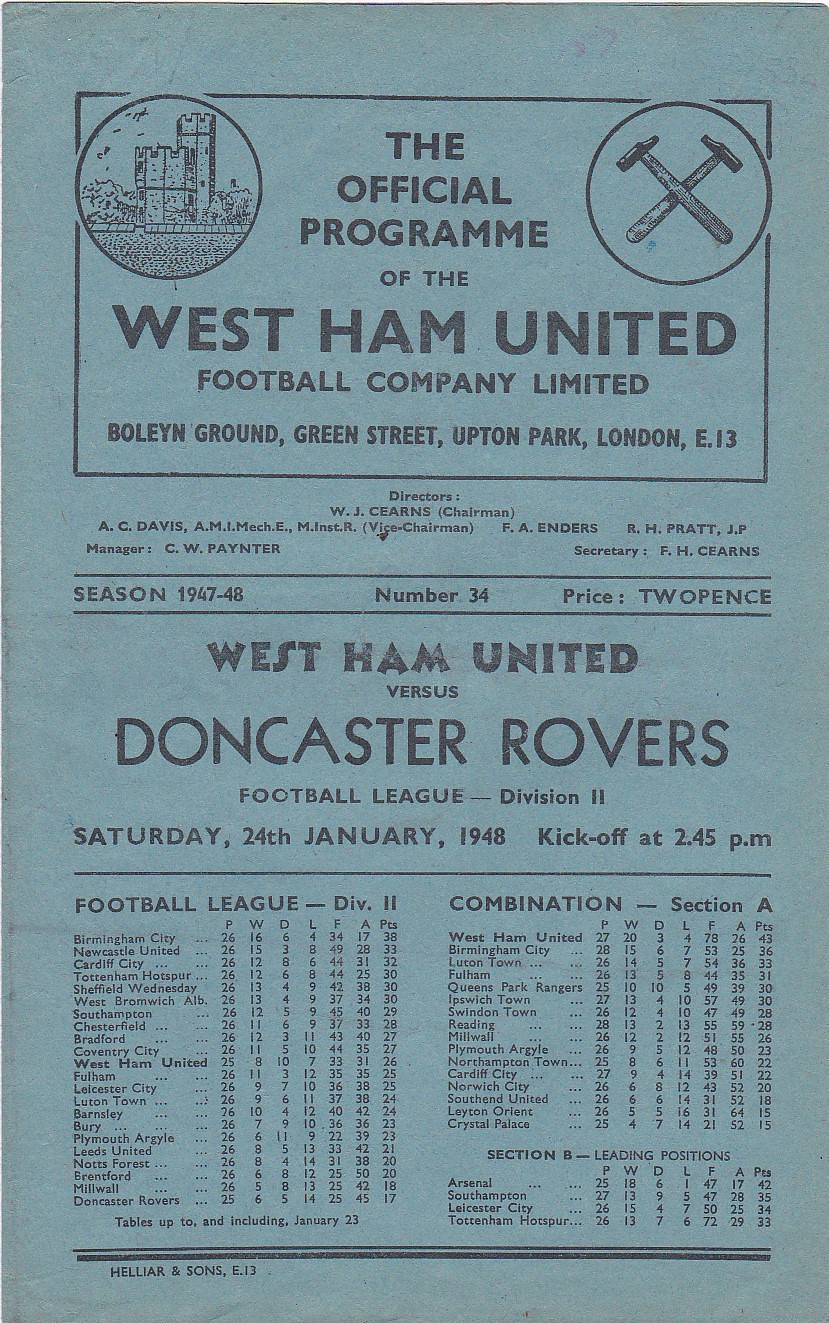This image depicts the official program of the West Ham United Football Company Limited for the 1947-1948 season. The cover is predominantly blue-gray with black text. At the top, a rectangular box contains several elements: on the left, a castle emblem inside a circle; on the right, two crossed hammers within a circle. The text within this box reads, "The official program of the West Ham United Football Company Limited, Bolin Ground, Green Street, Upton Park, London, E13." Below this are smaller, unreadable words, followed by larger text that states, "Season 1947-48, Number 34, Price 2 pence." Further down, it details the match information: "West Ham United vs. Doncaster Rovers, Football League, Division II, Saturday, 24 January 1948, kickoff at 2.45 p.m." Following this, the cover also mentions "Football League, Division II, Combination, Section A" and includes likely win/loss records and scores in two columns on standing of the football league and the combination section, although this part is too small to read clearly. At the bottom appears the name "Hellam & Sons" or possibly "Heller & Sons."